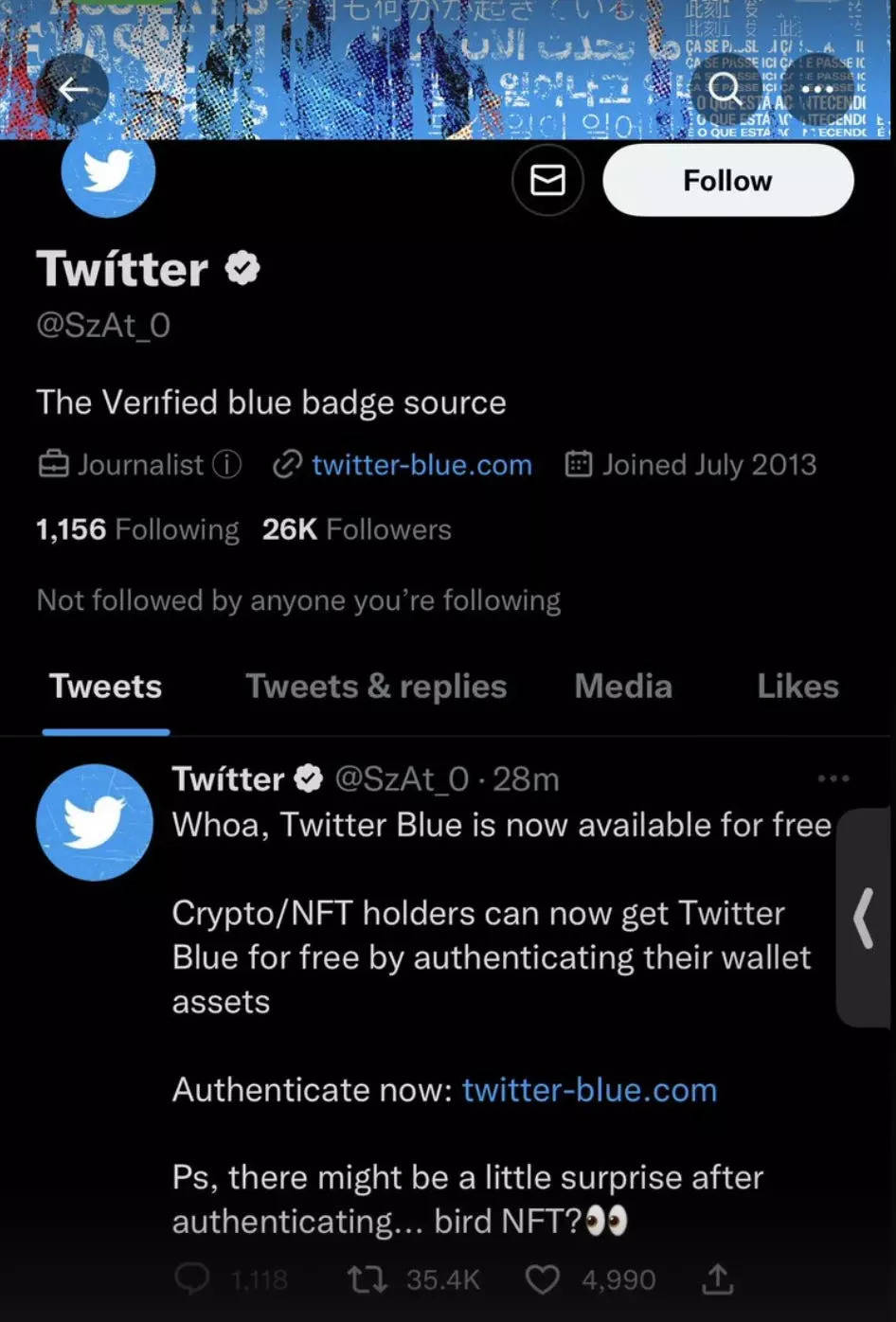This image is a screenshot displayed in portrait mode. The upper section, spanning from the upper left to the upper right corner, features an artistic light blue design with various art deco elements. On the left side is a back arrow icon, while the right side houses a search bar with a search icon.

The top left corner prominently shows the Twitter icon, and towards the upper right side is a large white "Follow" button. Below this header, the account information is displayed: the account name "Twitter" with a verification badge, and the handle "@SZAT_zero." Additional details include the verified status as a journalist via Twitter Blue, the join date "July 2013," and follower metrics indicating 1,156 following and 26,000 followers. It's noted that this account is not followed by anyone you are following.

Below the account details, there are category tabs for navigating through Tweets, Tweets & Replies, Media, and Likes. The most recent tweet, posted 28 minutes ago, reads:

"Whoa! Twitter Blue is now available for free. Crypto NFT holders can now get Twitter Blue for free by authenticating their wallet assets. Authenticate now at twitterblue.com. P.S. There might be a little surprise after authenticating Bird NFT 🐦"

A comment follows with skepticism about the offer, stating: "That sounds scammy."